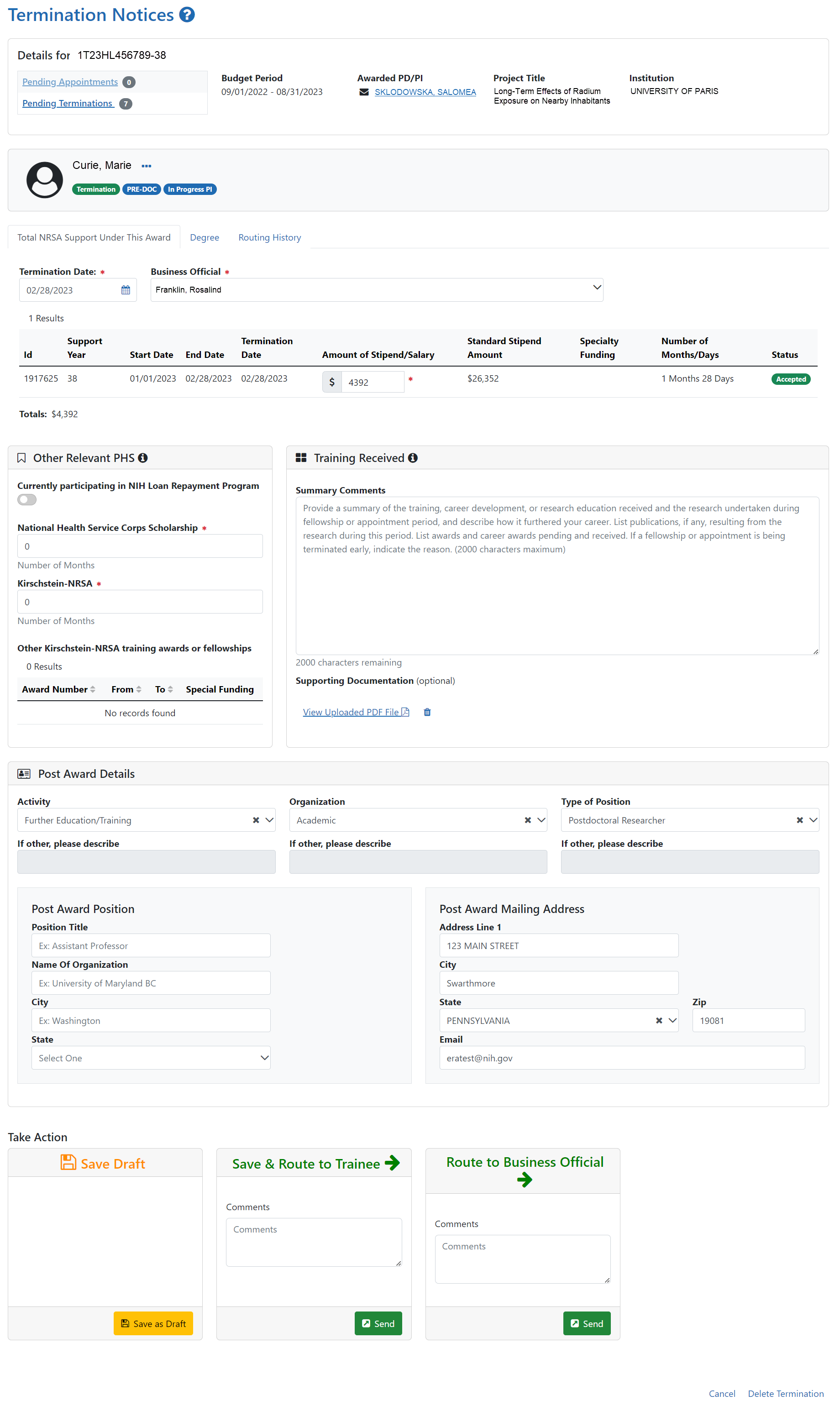Screenshot of a Website Showing Termination Notices for University Loans  

The image is a detailed screenshot of a website focused on termination notices. The background is predominantly white with various interactive boxes and text fields. At the top of the page, a blue header reads "Termination Notices." Below the header, there are several sections laid out in boxes.

In the first prominent box, titled "Details for Loan #XXXX," users can see clickable elements related to pending appointments, pending terminations, budget period, awarded PD/PI, project title, and institution. The institution listed here is the University of Paris.

Adjacent to this is another box with a placeholder for a photo, currently displaying a generic gray avatar labeled "Curie Marie." This section includes buttons for additional actions.

Further down, multiple boxes are arranged in a grid-like fashion. One box includes fields for termination date and business official, featuring interactive elements such as a calendar picker and a drop-down menu with names.

Another central box lists information such as ID, support year, start date, end date, termination date, and stipend/salary. Additional boxes provide details on other relevant PHS, training received, post-award details, post-award position, and post-award mailing address.

Towards the bottom, three boxes prompt users to "Take Action." The detailed layout concludes here, providing a comprehensive overview of loan termination information for users at the University of Paris.